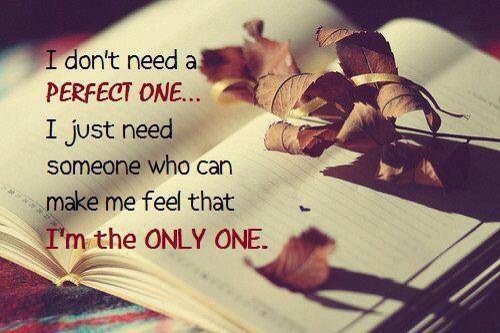This professionally shot, inspirational graphic features an open, blank journal with lined, beige pages and delicate embroidery around the edges, lying on a multicolored blanket. Dried autumn leaves and flower petals, casting soft shadows, are artistically scattered across the pages, adding a warm, yellowish glow to the scene. To the left of the journal, a motivational quote is prominently displayed in black and red text: "I don't need a perfect one. I just need someone who can make me feel that I am the only one." The image evokes a cozy, autumnal feel and is ideal for sharing on social media or a personal blog.